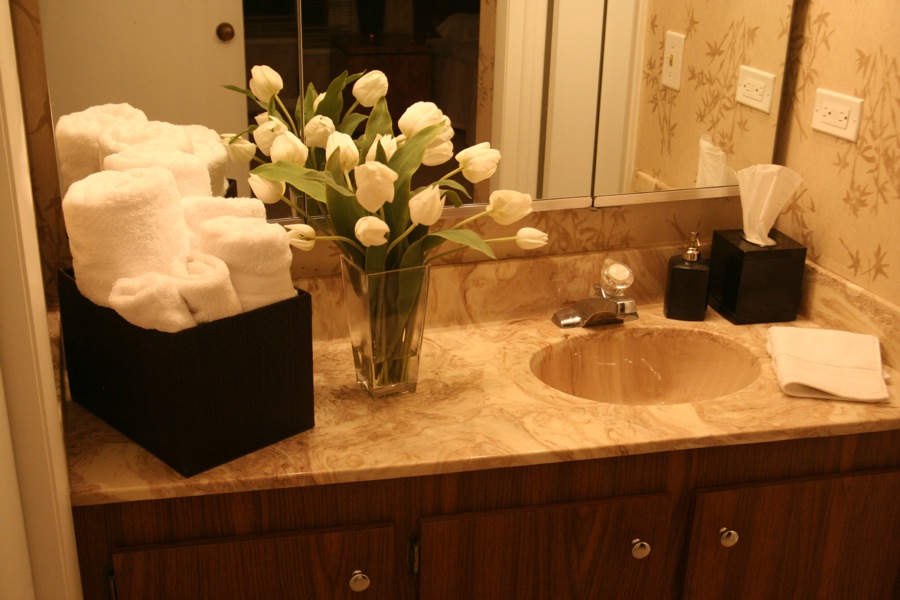A glimpse into an opulent bathroom, possibly belonging to a fancy restaurant or more likely a luxurious hotel. Dominating the space is a large rectangular mirror that reflects the image of a closet with sleek white sliding doors. The countertop, a stunning blend of white and brown marble, is adorned with a sophisticated ensemble: a black and silver soap dispenser, a black tissue box with a single tissue, a black basket filled with several neatly rolled white towels, and a clear rectangular vase brimming with white roses. To the side, an electrical outlet discreetly offers its convenience. The wall's subtle elegance is enhanced with a delicate floral design in brown. Below the countertop, richly-hued dark wood cabinets with silver handles complete the refined aesthetic.